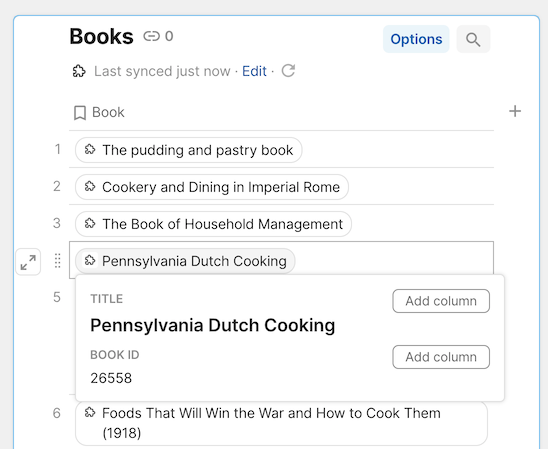The image showcases a neatly organized UI on a white background, bordered by a light blue outline on the top and sides, transitioning to a light gray outer border. In the top left corner, the interior space remains white, featuring the word "Books" prominently in large black letters. Adjacent to this, a small gray circle encloses a line and a zero. On the right side, a blue-shaded banner emblazoned with the word "Options" in blue is juxtaposed next to a gray-shaded square containing a gray search icon.

Below the "Books" header, a note states "Last synced just now" in standard text, followed by an "Edit" option in blue. Underneath this section, the word "Book" appears, separated by a fine gray line. Towards the far right of this segment, a plus sign is positioned to add new entries, divided by another fine gray line.

The section below lists six titles, each encapsulated in its own gray-shaded banner or outline. The entries are as follows:
1. "The Pudding and Pastry Book"
2. "Cookery and Dining in Imperial Rome"
3. "Book of Household Management"
4. "Pennsylvania Dutch Cooking" in a gray shaded banner
5. The text "Pennsylvania Dutch Cooking" reappears, followed by the "Book ID: 26558" and two adjacent banners labeled "Add Column".
6. "Foods That Will Win The War and How to Cook Them (1918)", outlined in a light gray banner.

The organized elements and neatly sectioned entries suggest a catalog or managerial interface intended for handling book titles and their details efficiently.